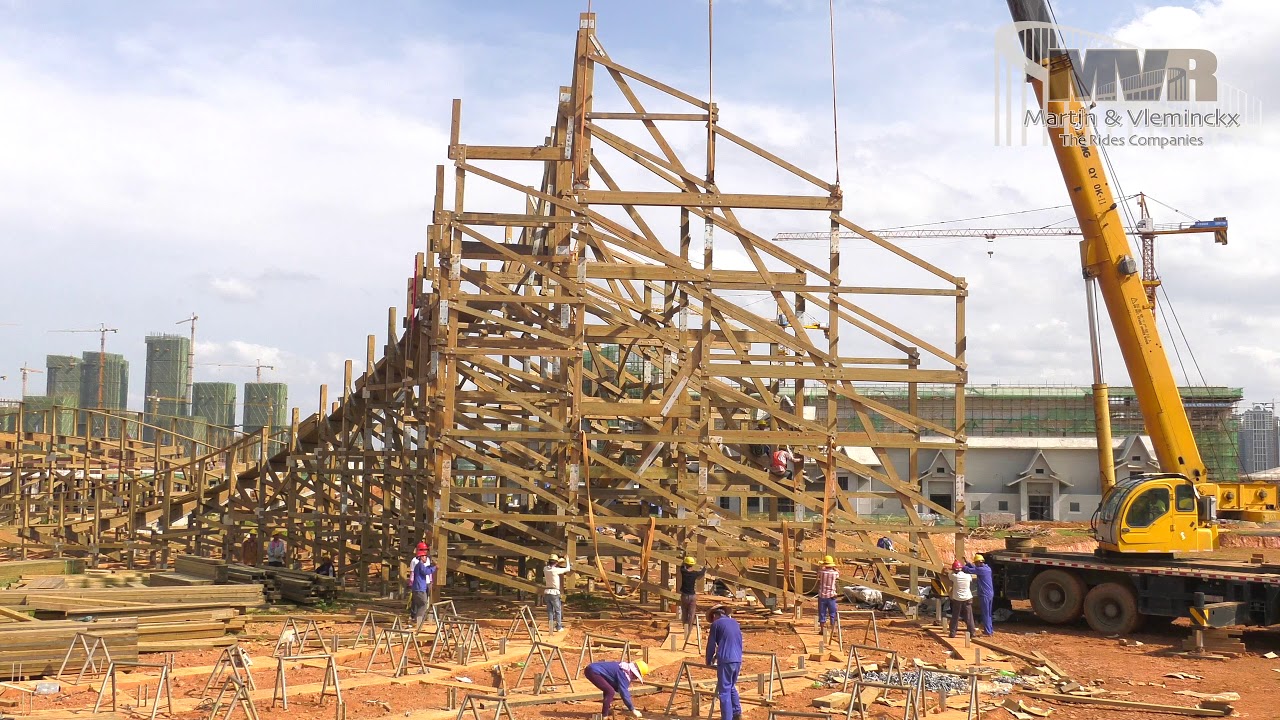The image depicts a bustling construction site, likely captured by the company MVR (Martin & Vleminckx: The Ride Companies) and posted on their website, evidenced by a small company logo featuring a roller coaster encircling the text in the top right corner. The primary focus of the picture is the assembly of what appears to be a roller coaster, indicated by a towering stack of tan-colored beams or possibly wooden structures that reach as high as a giant yellow crane dominating the right side of the image. 

In the foreground, around eight workers are actively engaged in various tasks, all donning hard hats—mostly yellow, with a few red. Their activities range from bending over to inspect materials to putting pieces together, all amidst an array of seesaw-type wood structures and several sawhorses. The sky above is mostly blue with significant white cloud coverage, creating a soft backdrop to the scene.

In the background, a mix of tall buildings, which could be hotels, apartments, or possibly industrial buildings, can be seen to the right of the structure under construction and around the heavy machinery. Additionally, some buildings with white and glass facades contribute to the urban setting. The overall image gives a clear and detailed depiction of an industrious site, with workers entrenched in the complex task of assembling what looks to be an amusement ride structure.